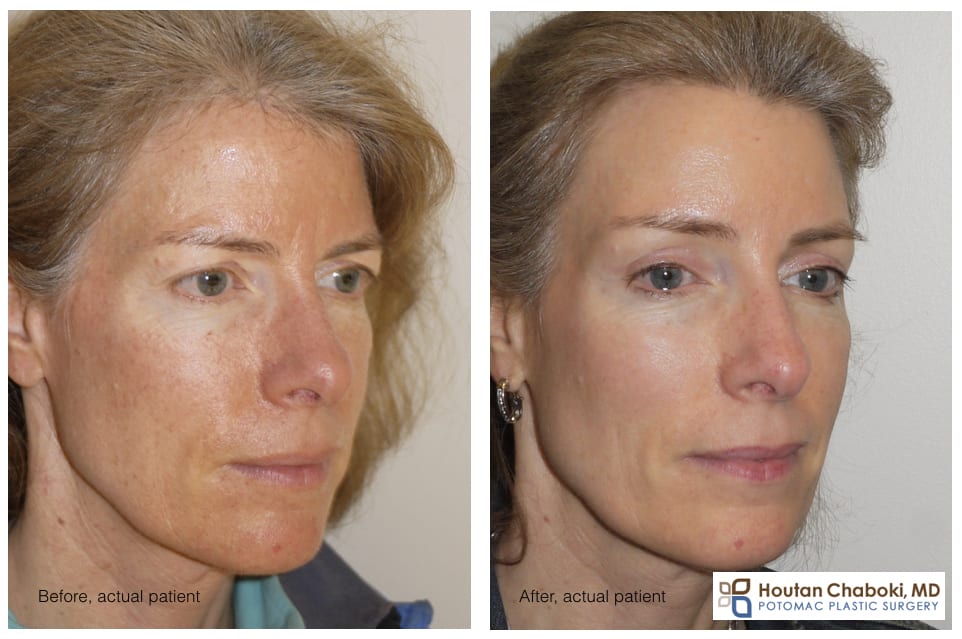The image depicts a detailed before-and-after transformation of an older woman, brought to you by Houghton Chibaki, MD, of Potomac Plastic Surgery. In both photos, she gazes somberly forward at a 45-degree angle, providing a clear view of her face and subtle changes. In the 'before' image, displayed on the left side, the woman's complexion is reddish-orange with noticeable melasma. Her white hair, with hints of brown and reddish tones, frames her face, which has an older appearance. She is dressed in an aqua-green shirt with a blue collar, and most of her left ear and the top of her head are cropped out of the picture. The text on the lower left corner reads "before, actual patient". In contrast, the 'after' image on the right reveals the same woman with a much-improved complexion—her skin appears smoother, more pink, and youthful, with the melasma significantly reduced. Her expression is almost a smile and she now sports an earring. Her bluish-green eyes appear brighter and more pronounced. This image also includes text at the bottom left "after, actual patient", and additional information in the bottom right corner identifying the plastic surgeon's name and specialty.